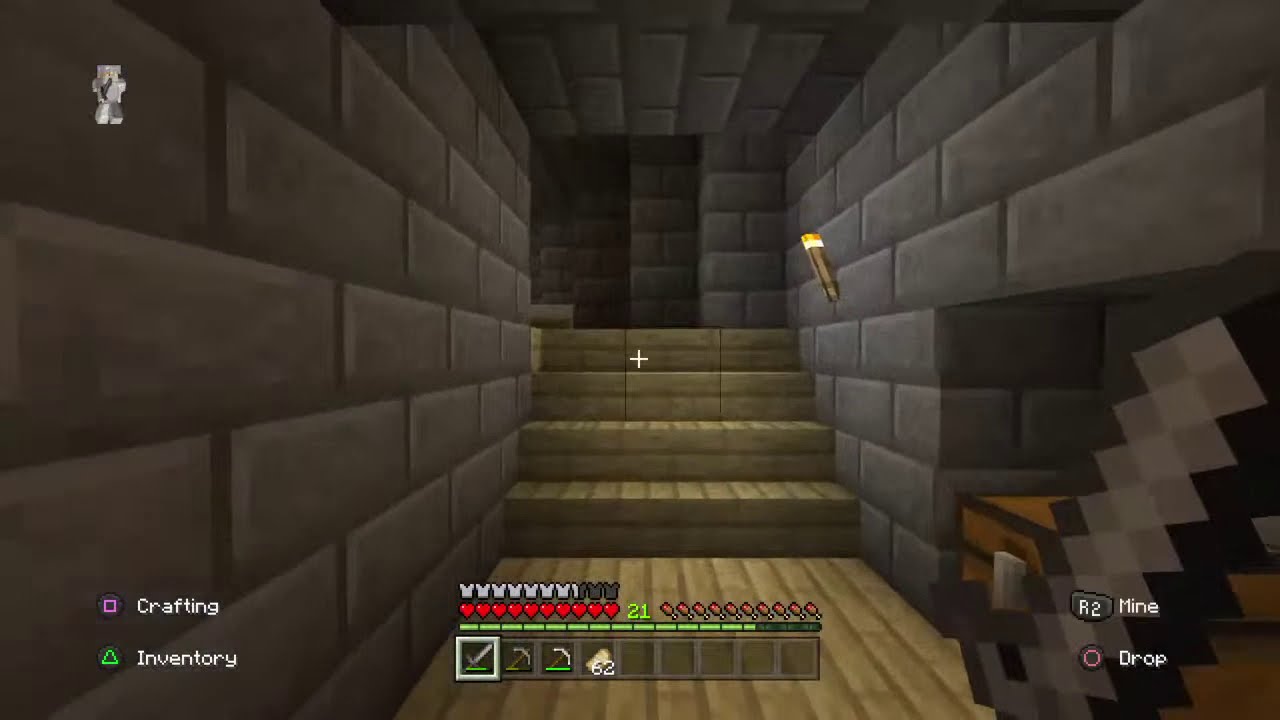This high-definition screenshot appears to be from a video game, likely Minecraft. It depicts an underground chamber or bunker-like setting with an immersive, cavernous ambiance. The scene is framed by gray brick walls on both sides and a matching ceiling. At the far end of this chamber are four yellow to light brown steps leading up to a corridor.

A torch is mounted on the right-hand wall halfway up the steps, casting a flickering light that brightens the immediate area. The floor contrasts with the walls, possibly made of a different material—a lighter tan or olive stone.

The user interface elements are prominently displayed. In the bottom left corner, there is the text "Crafting" with a small purple square icon and "Inventory" accompanied by a green triangle icon. The bottom center of the screen displays player status indicators including heart shapes representing health and possibly a green progress bar showing the number 21, which might indicate the player's level or progress in the game. Additionally, there are instructions for game controls: "Crafting" linked to the square button, "Inventory" to the triangle button, "Mine" associated with the R2 button, and "Drop" with the circle button. The entire image provides a comprehensive snapshot of the game's interface and environment setup, immersing the viewer in the game's atmosphere.